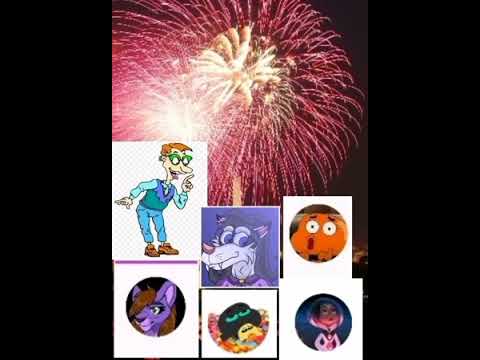The image features a black background with two vertical black stripes on either side, emphasizing the central focus. At the top of the image, vibrant fireworks explode against the dark sky. The fireworks display predominantly consists of red and white colors, with bursts of orange, violet, pink, and gold sparks radiating outwards, creating a luminous spectacle. 

Below the fireworks, there are six small, cartoonish illustrations arranged in a grid with a white background. In the top row, from left to right, the first image depicts a man with striking red hair, wearing green glasses, a blue outfit, brown shoes, and pointing to the left; he resembles the dad from Rugrats. Next to him is a dog dressed in a purple background, characterized by a white snout and purple fur. The third figure in this row is an orange cartoon character with white eyes and a red rectangle for a nose or mouth.

In the bottom row, the leftmost image shows a fox or a lion with purple fur and a brown mane extending from its head down its back. The center image is a stylized depiction of a fish-like creature, black with blue eyes and adorned with colorful flowers. The final image in this row is a girl encircled in a dark blue or purple border, dressed in a heavy blue coat with white trim, exhibiting black and white hair reminiscent of Cruella de Vil. The overall composition combines dynamic fireworks with whimsical cartoon characters, juxtaposing the lively outdoor scene with playful, illustrative details.